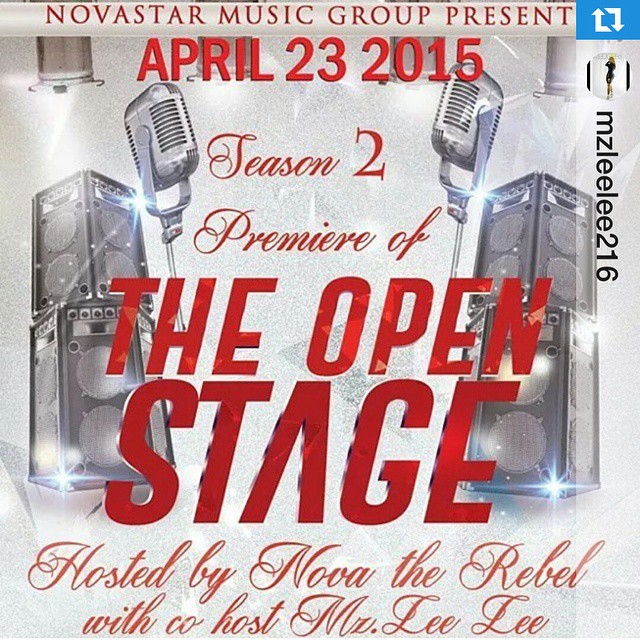The image features a poster promoting a concert event presented by Nova Star Music Group. At the top, in a smaller font, it reads "Nova Star Music Group present," followed by the date "April 23rd, 2015" in a larger, darker red font. Below this, the poster announces in cursive the "Season 2 Premiere" of "The Open Stage." The word "Stage" is styled with the letter 'A' resembling an upside-down 'V' and all the letters slanting slightly to the right. In cursive, it notes the event is "Hosted by Nova the Rebel with co-host Mr. Lee Lee," both in red cursive.

On each side of the text "Season 2," the background shows old-fashioned microphones, accompanied by stacks of two speakers each on both the left and right sides with spotlights illuminating them. Additionally, the right side of the poster features the label "MZLELE2116" written vertically in black.